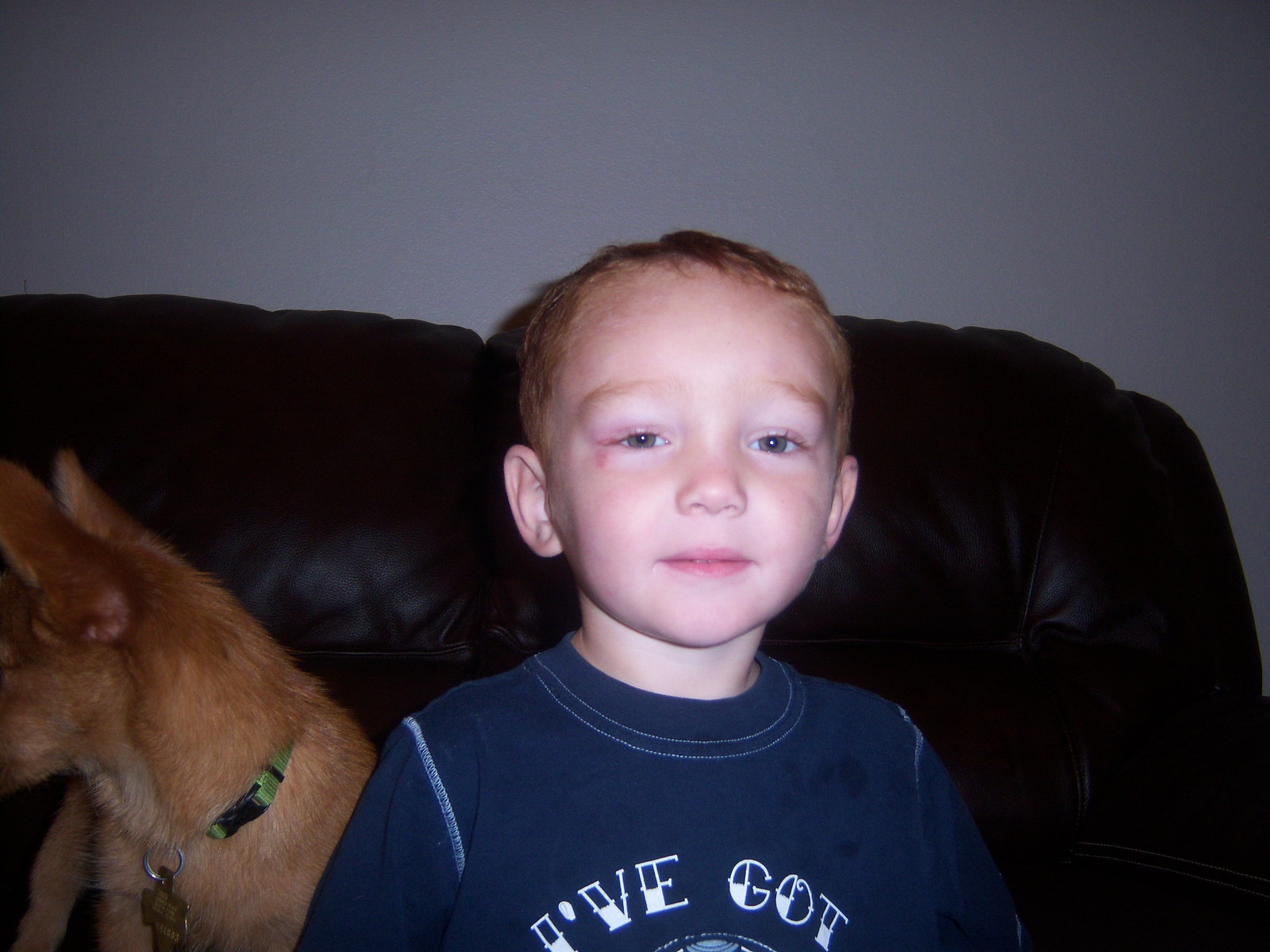This image captures a young boy, likely around four years old, with light blonde hair and fair skin, wearing a blue shirt that partially reads "I've got." He appears to have a noticeable mark and some swelling under his eye, possibly from a recent bump. The boy is seated on a dark brown leather couch, with a white wall in the background. Beside him is a small brown dog with a green collar featuring a gold tag. The dog's profile is visible, showing its ears but not its nose, as it looks away from the camera, seemingly distracted by something off-frame. The boy's shirt has a small stain on the shoulder, and a white ball can be seen behind him on the couch.